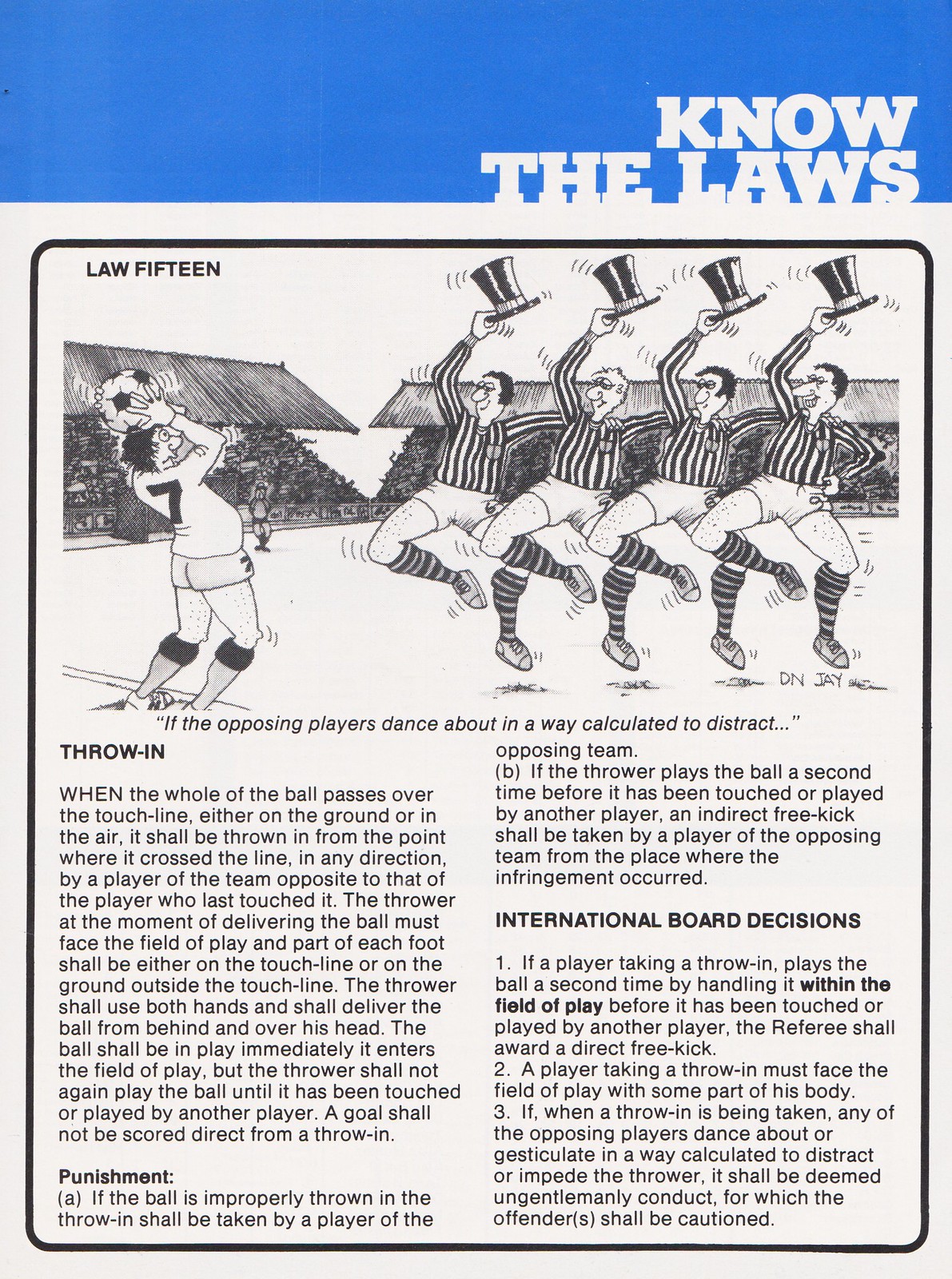The image is a vertical rectangular black and white poster with a prominent blue band at the top that reads "KNOW THE LAWS" in white letters. Below the band, the text in the upper left corner states "Law 15," indicating that the poster is about the rules surrounding the throw-in in soccer. Featured prominently in the center of the poster is a humorous, pencil-drawn cartoon scene. On the left side, a soccer player is holding a ball overhead, preparing to perform a throw-in. Opposite him are four figures dressed in referee uniforms; they are wearing white pants, striped socks, and top hats, and they are comically dancing in an attempt to distract the player. The characters are depicted with smiles and exaggerated expressions, adding to the comedic effect. Below the cartoon, detailed text explains the regulations and penalties associated with executing a throw-in incorrectly, alongside an interpretation of international soccer laws. Additionally, a quote at the bottom of the image mentions, "If the opposing players dance about in a way calculated to distract…", trailing off with an ellipsis to imply that such actions are considered a violation of the rules.